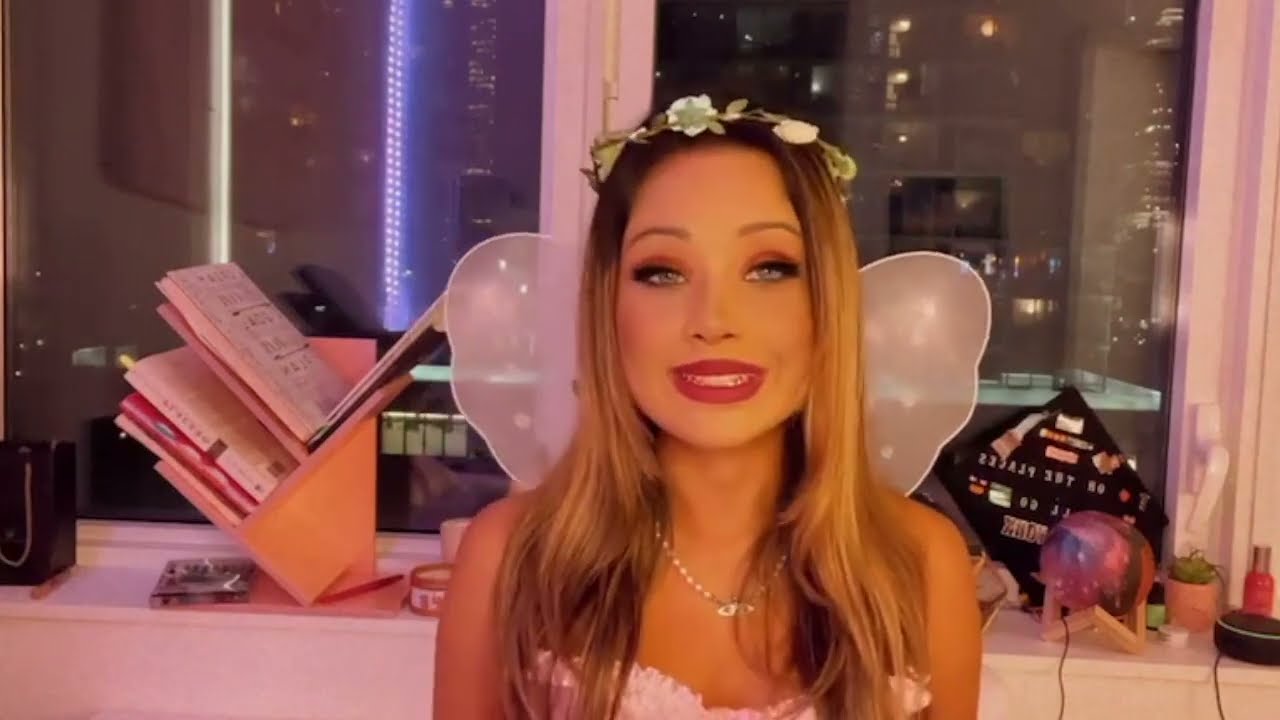In this image, we see a young girl dressed in intricate fairy cosplay, seemingly ready for a video blog or perhaps a Halloween outing. She is adorned with a flower crown made of leaves and twigs on her head, accentuating her long blonde hair with brown roots. Her makeup is striking, featuring red lipstick and blue eyes, though her smile appears slightly uncomfortable. She's wearing a pink dress and delicate pink fairy wings on her back, along with a notable pearl necklace around her neck.

The room has a whimsical ambiance, bathed in pink and purple hues. Various items are scattered across a windowsill behind her, including books, a DVD, a black diamond-shaped calendar, and a spherical mood light. An Alexa device is also visible. The window frames are white, providing a clear view of a nighttime cityscape with illuminated skyscrapers and apartment buildings. This scene is set in a high-rise building, with the backdrop of a bustling city adding context to her enchanting yet somewhat melancholy appearance.